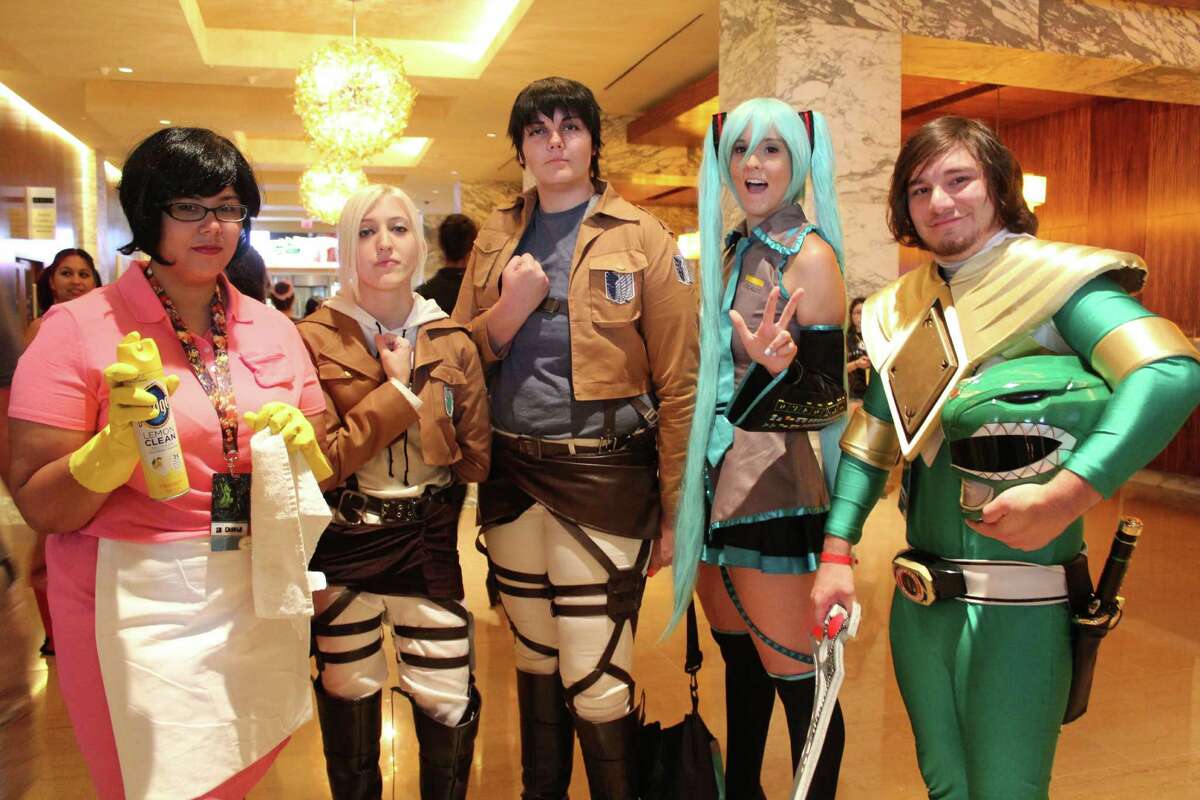This color photograph depicts a group of five young adults, likely between the ages of 18 and 22, standing in what appears to be a hotel lobby with yellowish-lit interiors. The group appears to be in cosplay, each donning distinct, vibrant costumes. On the far left, a lady with short, shiny black hair wears a bubblegum pink maid's dress, complete with a white apron, yellow gloves, and holding a yellow cleaning spray and a white towel, reminiscent of Rosalita from "Family Guy." Next to her, a lady with white straight hair is adorned in a brown jacket, white pants, brown leather skirt, and leather straps, with her hand placed over her heart. Beside her is a taller lady with black hair, wearing the same brown and white outfit and replicating the same hand gesture. Moving further, a woman with a striking long iridescent blue wig styled in knee-length pigtails sports a short skirt outfit. Finally, on the right stands a man with a goatee and long brown hair, wearing a bright shiny green jumpsuit that resembles a Power Rangers costume, complete with an elaborate gold shoulder pad and a dinosaur head helmet perched on the side.